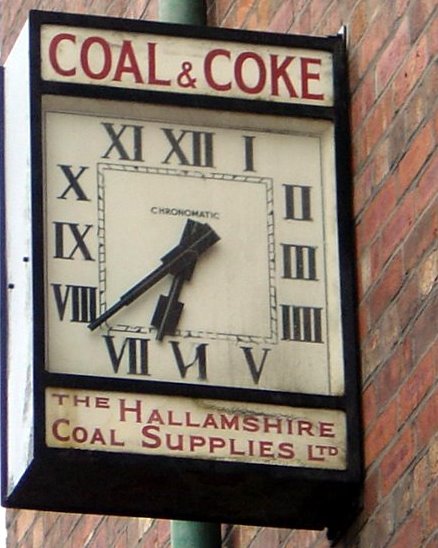In this outdoor photograph, the red brick facade of a building provides a striking backdrop to a prominently mounted clock. The clock, affixed to the short end of the building, stands out in its large, rectangular, three-dimensional frame. Above the clock face, a sign reads "Coal and Coke," while below, "The Halamshire Coal Supplies, LTD" is inscribed. The clock itself features a classic white face adorned with black Roman numerals and sleek, black, thin rectangular hour and minute hands. The combination of the clock's traditional design with the robust, industrial aura of the building offers a nostalgic glimpse into times gone by.